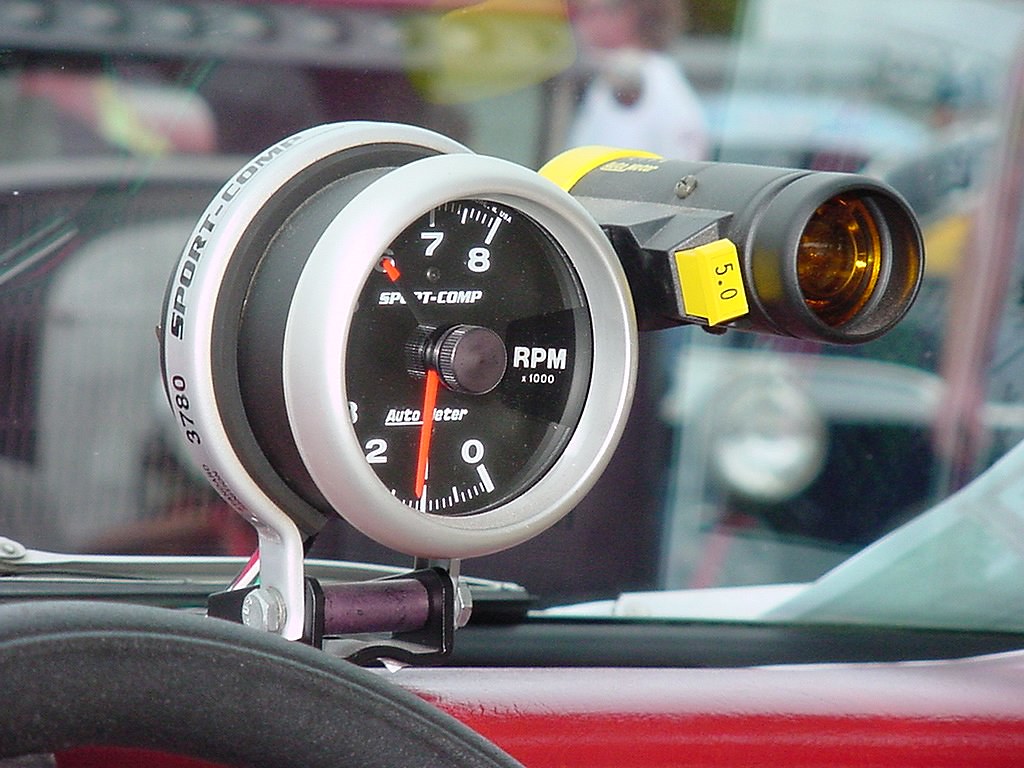This image showcases an altimeter situated inside a car with a striking red dashboard. The steering wheel is dark gray, and the windshield is made of clear glass, providing an unobstructed view. The altimeter itself is circular and gray with black trim and a black center. It features white letters and numbers with red dial hands. Prominently displayed at the top of the altimeter are the numbers 6, 7, and 8, while the numbers 3, 2, 1, and 0 are visible at the bottom. The center of the altimeter is labeled with the words "ALTIMETER Sport Comp, RPM x 1000." Encircling the edge, it reads "3780 SPORT COMP." Positioned at the top right side of the altimeter is a darker gray cylinder with an amber lens, marked by a small yellow tag that reads "5.0." For additional details, the tag includes a reference to www.Flydreamers.com.